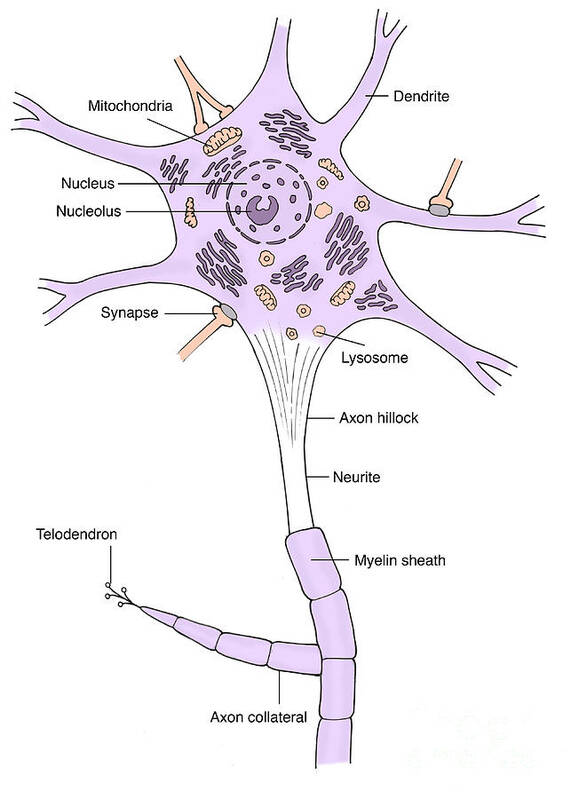The image depicts a detailed diagram of a motor neuron on a white background. The neuron is primarily illustrated in black line drawing with elements shaded in light purple and brown tones. At the top of the diagram, a purple splotch representing the dendrite extends into six arms, leading down through a white 'neck' into another segmented purple tube. This tube, which also has an offshoot to the left, features multiple labels identifying various cellular components.

Starting from the left offshoot, labeled as the telodendron and axon collateral, the diagram further includes the myelin sheath enveloping segmental sections along the length of the neuron. The central area highlights the nucleus, a darker purple circle in the core, with the lighter nucleolus inside it. The surrounding structures include the mitochondria, depicted as pink squiggly lines, the lysosome illustrated as round circles, and synaptic ends shown as orange tubes.

Additional labels mark critical points such as the axon hillock and neurite, which serve as transitional regions between the main segments of the neuron, and the continuous structure of the myelin sheath that insulates the axon. Altogether, the diagram is a comprehensive visual representation of the intricate components within a motor neuron, each meticulously labeled to detail its specific cellular function.